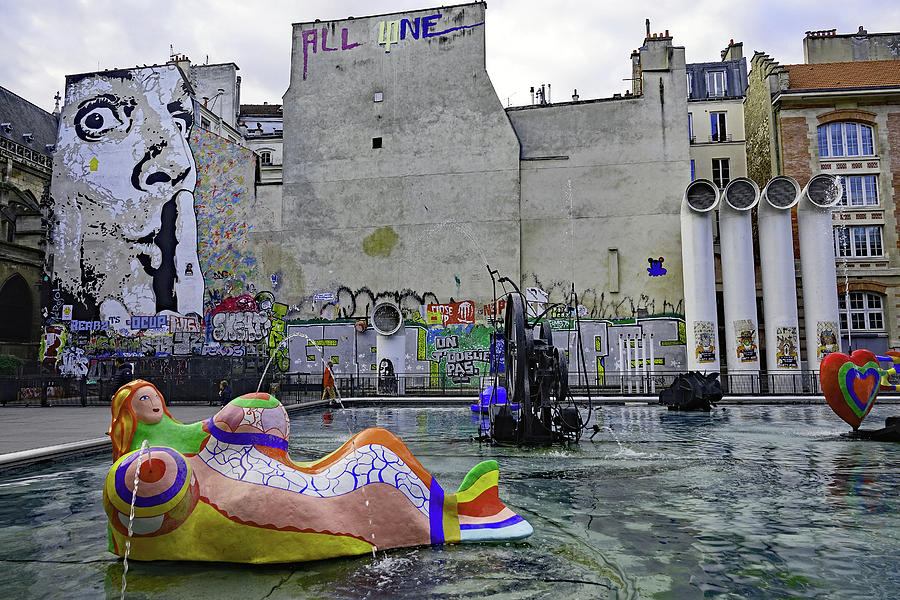The image depicts a downtown area featuring a water park with a shallow pond or fountain at its center. Dominating the foreground is a striking and abstract mermaid sculpture, multicolored, with pronounced, fountain-featured breasts spraying water. The scene is surrounded by various other stone and metallic sculptures, adding an artistic flair to the watery environment where one can imagine people leisurely strolling, as evidenced by a person in a red jacket visible in the background.

The surrounding architecture consists of several brick buildings, approximately three to four stories high, decorated with vibrant murals and extensive graffiti. Noteworthy is a large black-and-white mural on one building, depicting a wide-eyed man placing his finger to his lips in a shushing gesture. Tall, white pipes also rise in the background on the right-hand side, contributing to the eclectic urban aesthetic. Despite the artistic atmosphere, the area doesn't give off a particularly metropolitan or safe vibe, hinting at its character and age.